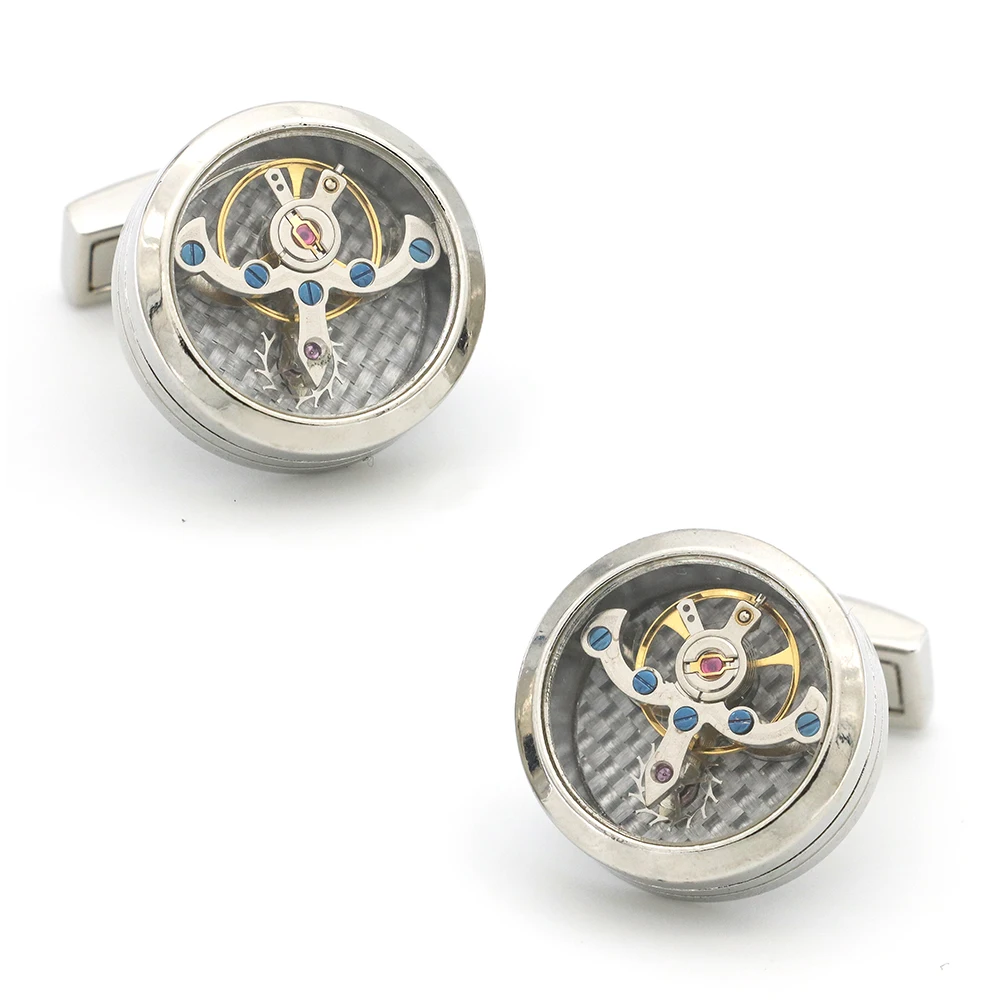The image depicts two identical silver cylindrical gadgets against a white background, each encased in see-through hollow metal featuring a sophisticated design. The devices consist of a flat circular clear container, likely with a layer of glass on top, secured with five blue screws across the middle and a purple gem at the bottom, surrounded by a spiral of metal. A red gem encased in gold is situated near the top, further emphasizing the intricate design. Inside, a gold circular ring is visible, with an element resembling an airplane—complete with plane wings and a nose—situated on top. Extending from the airplane-like piece is a spiky silver reed. Both gadgets have a shiny, stainless steel-like appearance, and are displayed almost facing each other: the one on the left is positioned upward, while the one on the right is positioned downward and slightly ajar. They possibly serve a functional purpose, perhaps telling time, and are laid out on a pristine white backdrop, enhancing their metallic sheen and detailed craftsmanship.